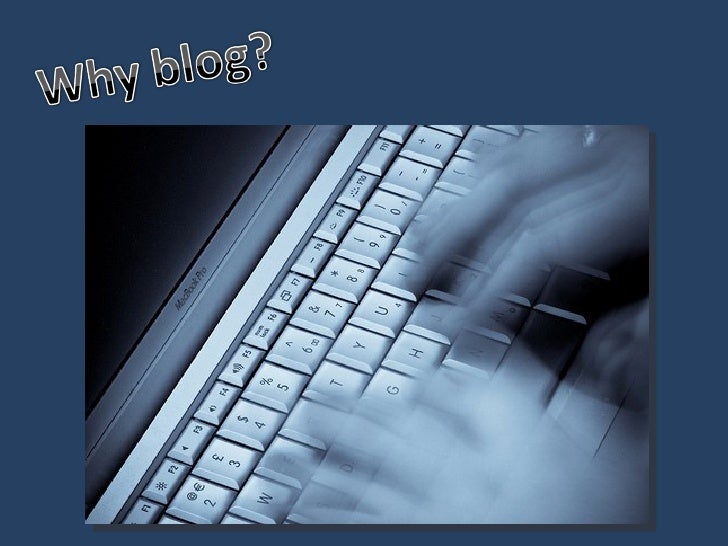The image depicts a close-up of rapidly typing hands on a MacBook Pro keyboard at a slight diagonal angle. The hands, emerging from the right side of the image, are blurred due to the speed of typing. The keyboard, tilted with a white finish, displays labeled keys and is identified as part of an older MacBook Pro model situated just beneath the screen. The backdrop features a large blue frame that narrows towards the bottom, enveloped by a substantial gray border on the left, top, and right. Black, white, and gray text positioned above the image reads "Why Blog?" in an old-school, shiny 3D font, though slightly tilted. The professional composition of the image suggests it could be used in a slideshow or on a website to emphasize the importance of blogging.